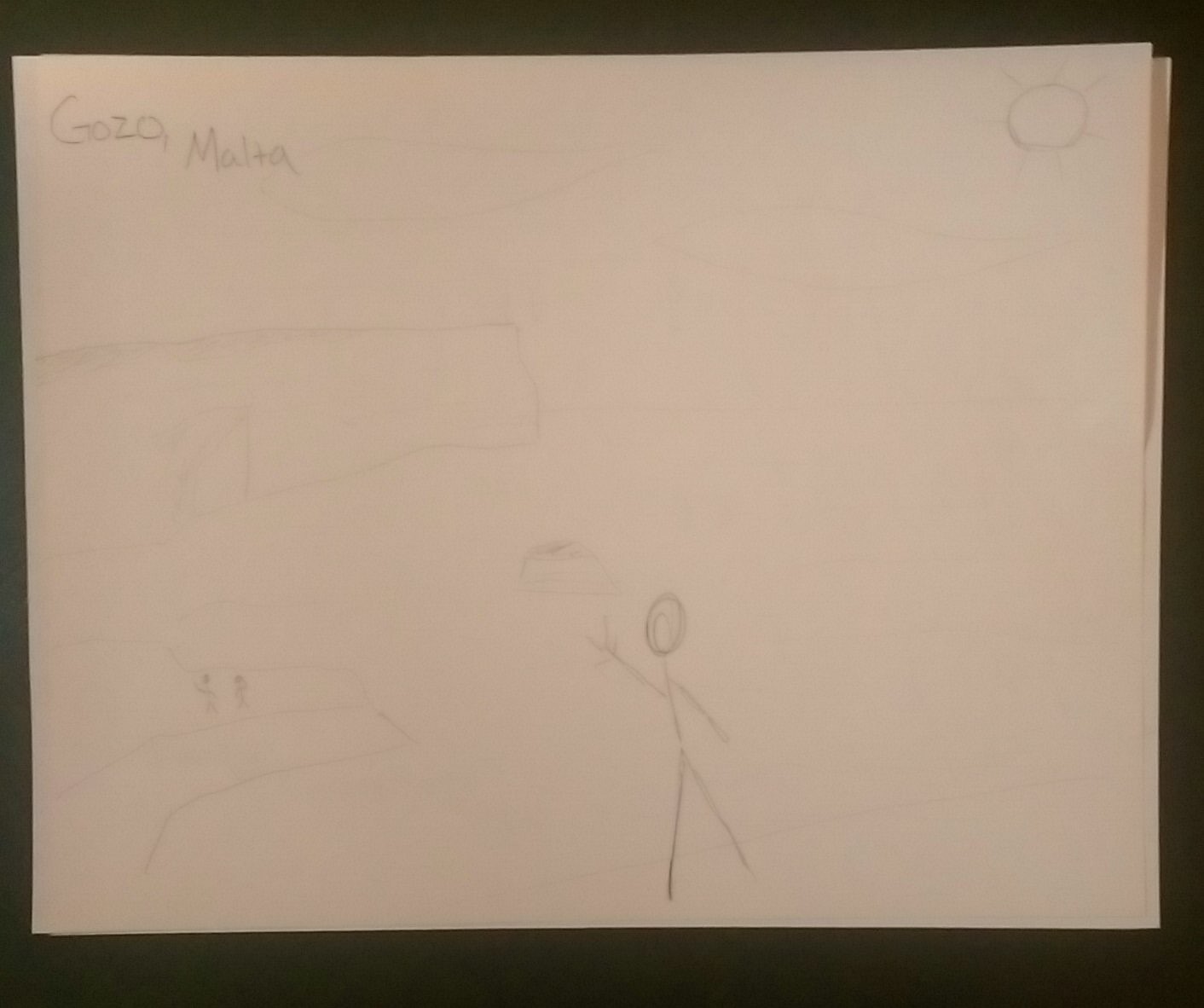This photograph is of a pencil drawing on a slightly pink-toned piece of paper. In the top left corner, the text "G-O-Z-O, M-A-L-T-A" is faintly visible, and in the top right, there is a sketch of a sun represented by a circle with lines radiating from it. Centered at the bottom of the paper is a stick figure, characterized by a circle for a head, a simple line for a body, two lines for legs, and stick arms with three fingers on each hand; one of these arms is raised as if waving. To the left of this main stick figure, some faint lines hint at additional elements, including two smaller stick figures that seem to emerge from a divided rectangular shape, adding a subtle complexity to the simplistic scene.